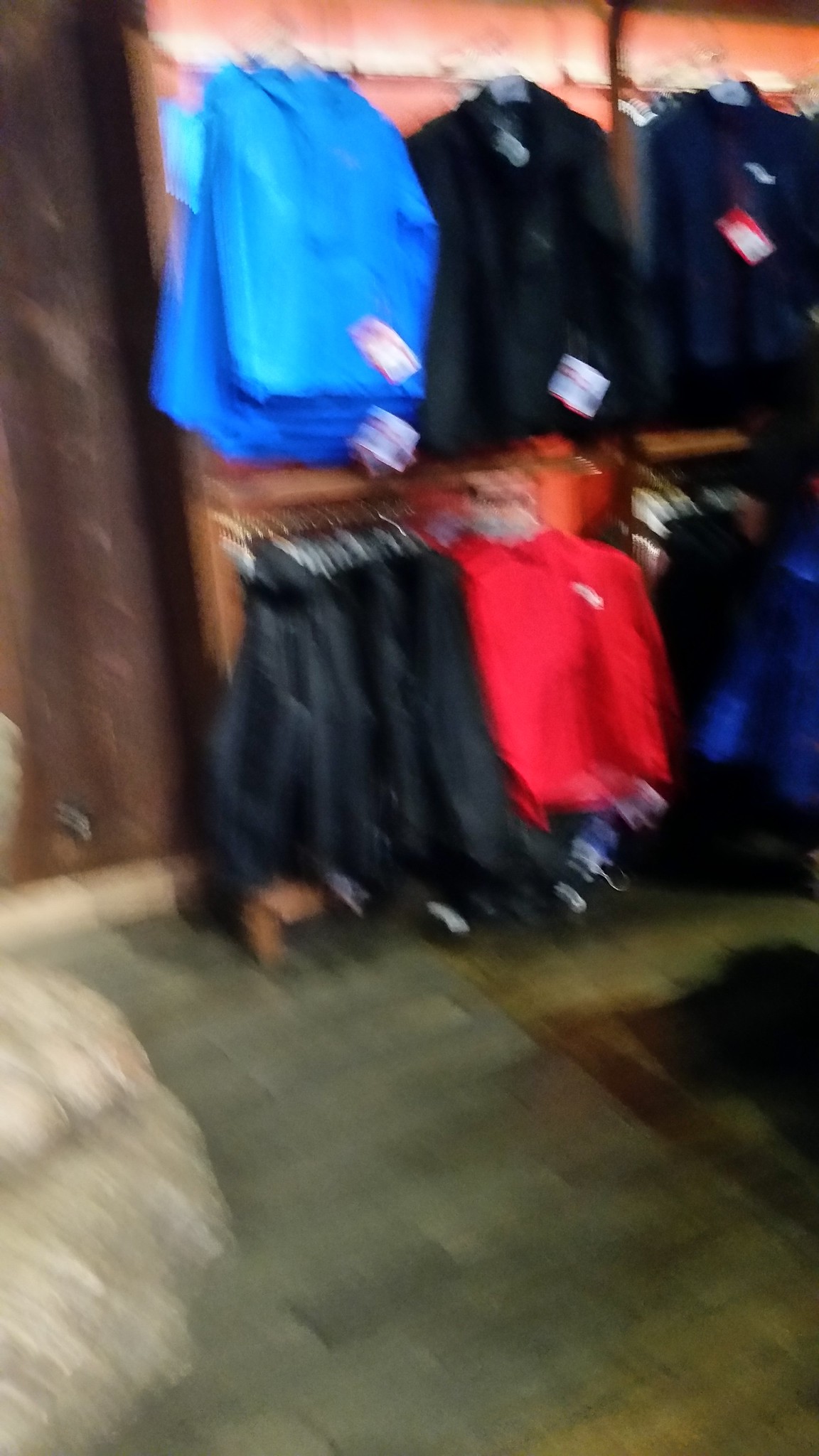The image depicts the interior of what appears to be a department store. The scene is slightly blurry, but the arrangement and variety of garments on display can still be discerned. Along the wall, there are two rows of clothing racks. On the top left, a stack of bright blue shirts is prominently visible. To their right is a cluster of black shirts, followed by dark blue shirts adorned with red labels.

On the bottom left rack, a selection of what seems to be black leather jackets is displayed. Adjacent to these are red shirts, followed by alternating black and blue shirts. The flooring is covered with greenish carpet, contributing to the store's subdued ambiance.

To the left of the clothing racks, a wooden door is noticeable, adding a rustic touch to the otherwise modern setting. At the bottom left corner of the image, there is an indistinct object that appears to be made of glass or plastic, though its features are difficult to discern due to the image's blur.